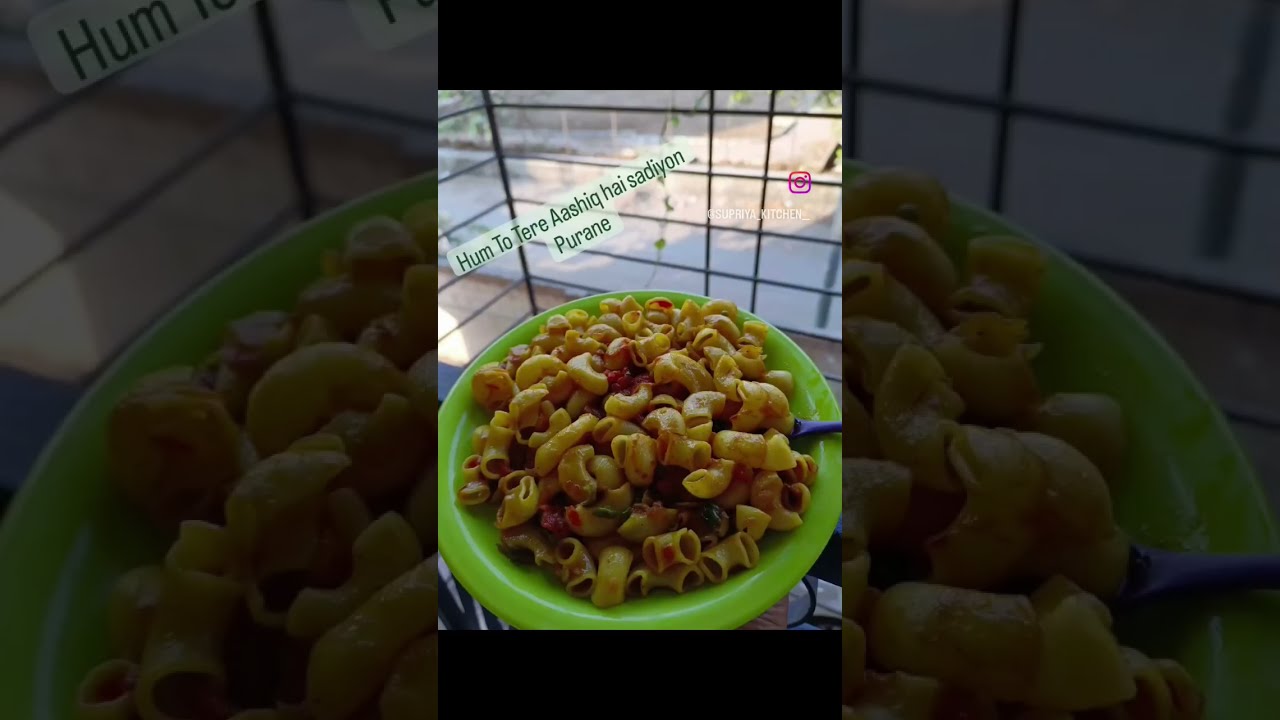This image, resembling a mobile phone screenshot, captures a photo of a vibrant food dish, prominently featuring macaroni pasta stir-fried with tomatoes and green chilies, garnished with herbs. The macaroni sits inside a neon green bowl, with a blue spoon extending from it. This setup is positioned against a background that suggests an indoor or balcony setting, evidenced by the visible metal frame. The lower part of the background displays a blurred garden view or street scene, indicating depth and an outdoor perspective.

The image is divided horizontally with black rectangular blocks at the top and bottom, giving it a distinctive framed look. On the upper right corner, the Instagram logo is visible, affirming its social media origin. To the upper left, there are foreign text inscriptions: "hum2teaashiq, H-A-I-S-A-D-I-Y-O-N," and below, "purane, P-U-R-A-N-E," likely adding cultural context. A pink camera icon appears next to a handle, "at Supriya underscore kitchen." On either side of the central photo of the macaroni bowl, enlarged and darkened halves of the same image are placed, creating a triptych effect.